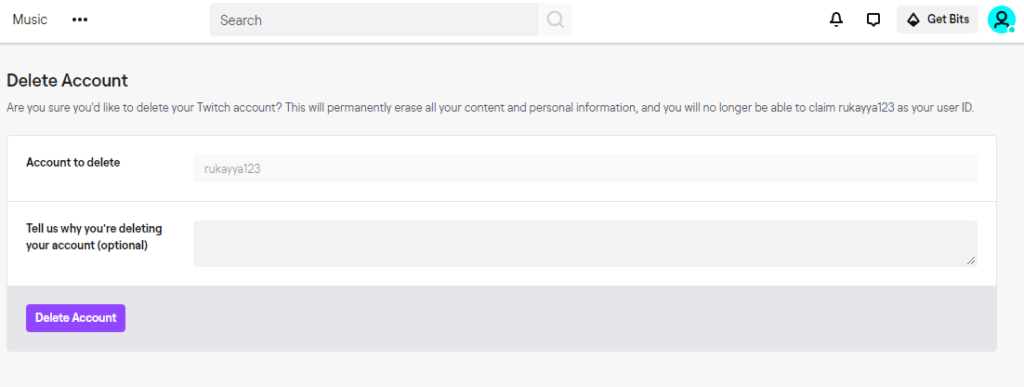The image depicts a user interface, likely of a mobile or web application, focused on deleting a social media account. 

In the top left corner, the word "Music" is prominently displayed. Nearby, three identically-sized horizontal dots are aligned, suggesting additional settings or options. Adjacent to these dots is a gray search bar labeled "Search," complete with a magnifying glass icon on its right side for activating the search function. 

On the top-right corner of the interface, a series of icons are lined up: a bell icon for notifications, a speech bubble icon for messages, and a diamond-shaped icon labeled "Get Bits." Further to the right is a teal-colored circle featuring a person icon, accompanied by a small dot in its bottom right corner, indicating a possible new notification or message.

Below this header, a gray rectangular bar features the bold text "Delete Account." Directly beneath this, the text "Are you sure you'd like to delete your Twitter account? This will permanently erase all your content and personal information and you will no longer be able to claim RUKAYYA123 as your ID" is displayed in gray.

A white box is centrally positioned, divided into two sections. The upper section, titled "Account Delete," contains a gray box where the username "RUKAYYA123" has been entered. Below this is a prompt asking "Tell us why you are deleting your account," which is marked as optional in bold type. A large gray text box is provided for the user’s response.

At the very bottom, a gray bar of the same width as the white box presents a purple button labeled "Delete Account."